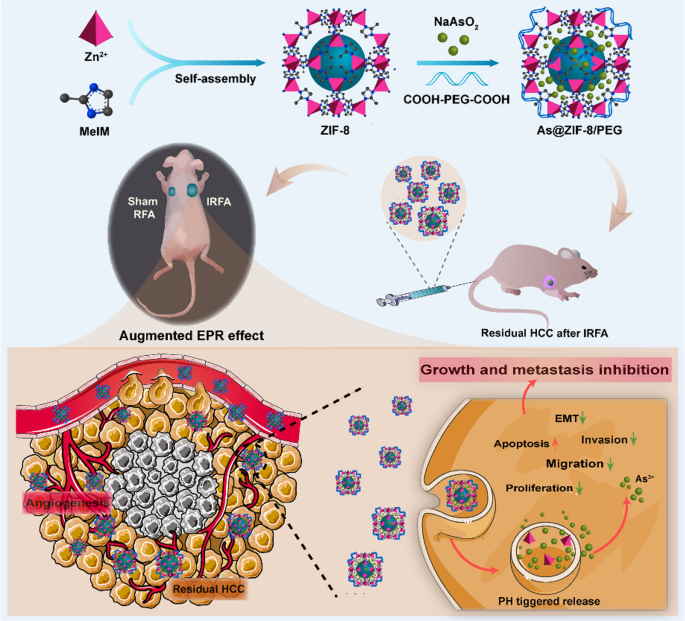This detailed scientific diagram is a colorful cartoon-style illustration divided into two main sections. The top half has a background of light blue and features an overhead view of a white mouse within an oval circle labeled "sham RFA" on the left side and "IRFA" on the right, indicating different experimental conditions. There is also a side view of a mouse with a syringe positioned nearby, labeled "residual HCC after IRFA," showing where the residual hepatocellular carcinoma (HCC) remains after the treatment. Surrounding the mice are numerous scientific notations, including DNA helices, elemental symbols like NA, AS, O2, and ZN2+, and terminologies such as "augmented EPR effect" and "self-assembly."

The bottom half of the image is a detailed representation of the internal dynamics of a tumor. The lower left section features depictions of yellow circles with silver centers, outlined in red, labeled "angiogenesis, residual HCC." The adjacent right section explains mechanisms to inhibit tumor growth and metastasis with several key terms like "pH-trigger release," "proliferation," "migration," "invasion," and "apoptosis." Green arrows in a peach-colored drawing further illustrate these processes, emphasizing the inhibition of growth and metastasis. Additional annotations include "EMT" and details of how the medication impacts these cellular activities. Overall, the diagram is a comprehensive visual representation of how a specific medication can inhibit the progression and spread of cancer in a rat model.